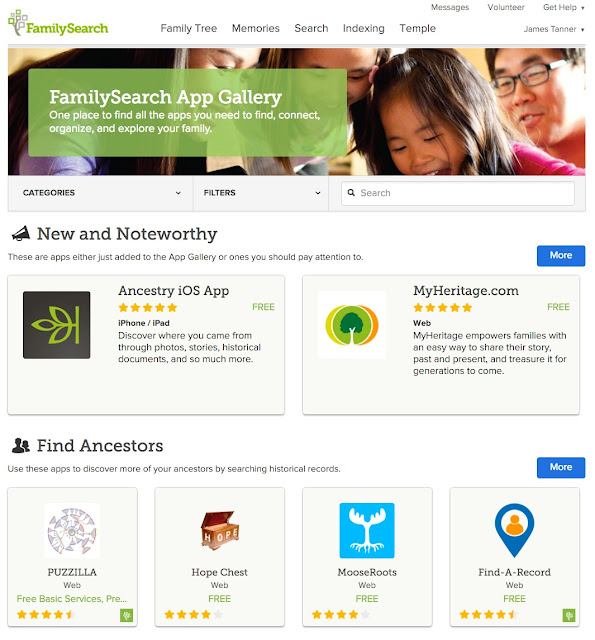A screenshot from the FamilySearch website is presented with a predominantly white background. In the upper left-hand corner, the green FamilySearch logo is prominently displayed. To the right, various navigation tabs appear in gray, labeled as Family Tree, Memories, Search, Indexing, and Temple.

In the upper right corner, additional options are visible, including Messages, Volunteer, and Get Help. Directly below this menu, the name "James Tanner" is displayed, presumably the logged-in user.

The main section of the image features a photograph of an Asian family looking downward. The mother’s face is partially obscured by a green overlay box. The father, wearing black glasses, can be seen in the background. The green overlay prominently features the text "FamilySearch App Gallery" in white, along with a tagline: "One place to find all the apps you need to find, connect, organize, and explore your family."

Below the image, the website sections labeled Categories and Filters are shown next to a white search box featuring a black magnifying glass icon. Further down, in black text, the headline "News and Noteworthy" indicates that the apps listed are either newly added or particularly significant. The first highlighted app is the "Ancestry" iOS app for iPhone and iPad, followed by "MyHeritage.com," both rated with five stars.

A section titled "Find Ancestors" suggests various apps for discovering ancestral records. Listed apps include Puzzilla, Hope Chest, Moose Roots, and Find a Record Web.